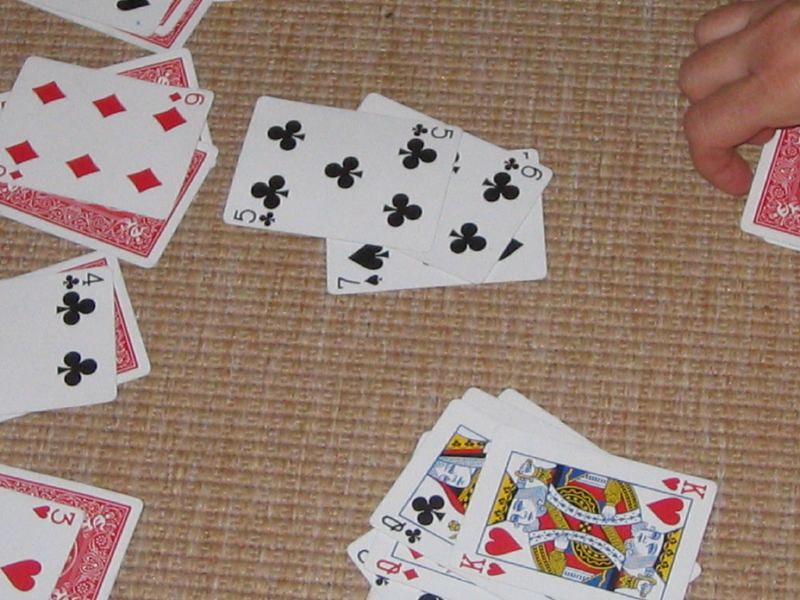In this image, we see someone deeply engrossed in a game of cards, set against a backdrop of a textured, woven carpet that covers the entire scene. The carpet features a rich blend of tannish-brown hues interspersed with specks of gray and tan, creating a visually engaging pattern that offers a tactile feel. In the upper right-hand corner of the frame, a partially visible hand—three fingers curled around the knuckles—holds several red-backed playing cards. The player appears to be engaged in a solitaire game, evidenced by the arranged piles of cards.

The bottom right section of the image shows a neatly stacked sequence of queens and kings, indicative of the player's progress. Adjacent to it is a column of descending black cards—seven, six, and five—though they belong to different suits. Four piles of cards are prominently displayed: in the upper left corner, two red-backed cards face down with a black spade face up on top; the next pile features red cards beneath a six of diamonds; another follows with a red card below a four of clubs; and the bottom left pile reveals a face-down red card topped by a three of hearts. This meticulous arrangement offers a glimpse into the strategic gameplay, adding a layer of intrigue and engagement to the scene.